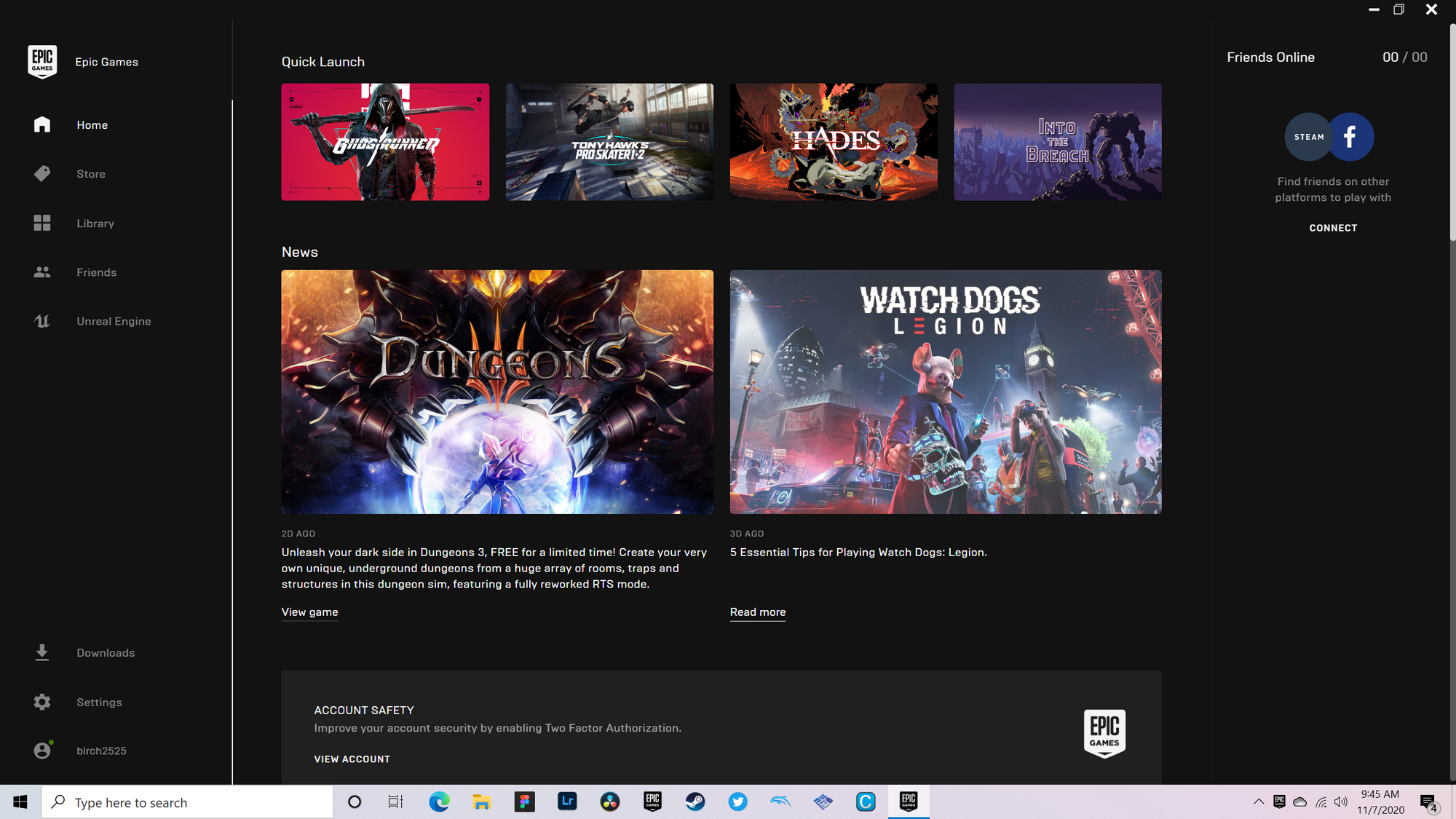This image appears to be a screenshot from a computer, displaying an Epic Games interface on a black background. At the top, there are quick launch icons, primarily featuring games. Images show characters in armor, with titles too small to read without zooming in.

On closer inspection from left to right: 
- **Tony Hawk**: A title related to Tony Hawk is visible but unclear.
- **Pro Slayer**: Faintly legible text suggests a game named "Pro Slayer".
- **Hay Days**: Another game title.
- **Into the Breach**: This game's icon depicts a monster standing on the edge of a cliff.

Beneath these:
- **Dungeons**: An image shows a monster peering into a crystal ball containing a person. Below this, text reads: "Two days ago, unleash your dark side in Dungeons, free for a limited time. Create your very own unique underground dungeons from a huge array of rooms, traps, and structures in this dungeon sim featuring a fully reworked RTS mode."
- **Watch Dogs Legion**: Depicts a mouse character in front of futuristic buildings. Accompanying text mentions: "Five essential tips for playing Watch Dogs Legion. Read more."

Additional elements include:
- **Account Safety**: A button for account safety measures.
- **Epic Games Logo**: Located in the lower right-hand corner.
- **Navigation Bar on the Left**: Includes sections like "Epic Games," "Home" (highlighted), "Store," "Library," "Friends," "Unreal," "Empire," and "Download Settings."
- **User Information**: The user identified as Bert2525.
- **Bottom Interface**: A white search bar, Windows logo, and icons on a grey background bar.

The overall layout and content indicate that this is a gaming site, specifically showcasing the Epic Games platform.